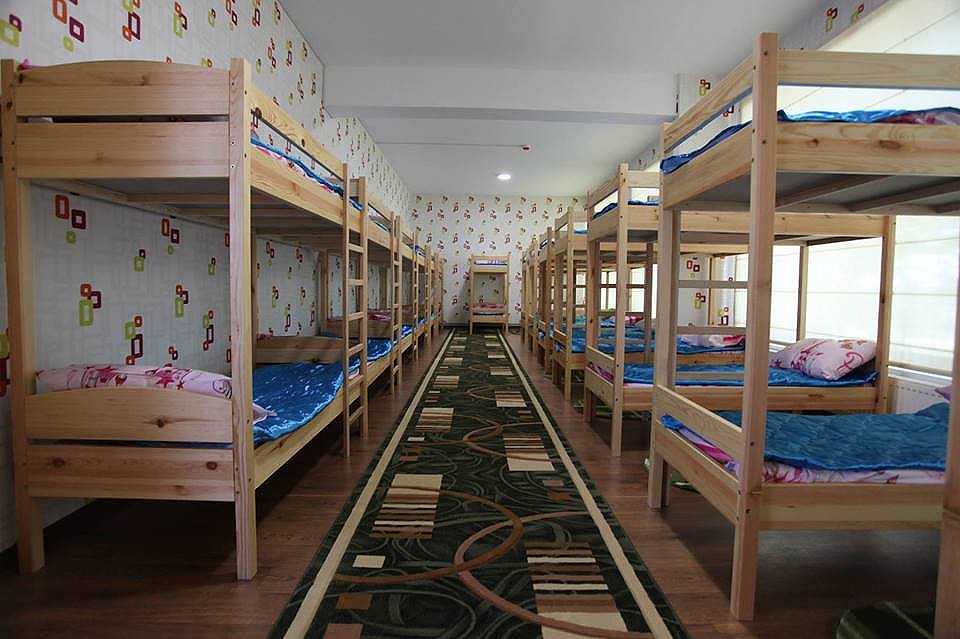This rectangular photograph, wider than it is tall, captures the interior of a long, narrow dormitory room lined with at least five sets of unfinished wooden bunk beds on each side. The beds are dressed uniformly with a solid royal blue quilt, underneath which lies a pink blanket. Each pillow, which appears to be pink with patterns or possible princess designs, adds a touch of whimsy. The room's floor is made of dark brown wood, complemented by a long, geometrically patterned runner rug in shades of green, brown, and beige running down the center.

The right wall features large windows while the left wall is adorned with off-white wallpaper decorated with geometric designs in green, purple, red, and beige squares. Ladders are affixed to each bunk bed, providing access to the top bunks. At the far end of the room, there's another wooden structure, appearing similar to the bunk beds but possibly serving as a bookshelf or cupboard, crafted from the same light-colored wood and featuring multiple colored panels in light brown, dark brown, cream, and green, adding a unique focal point to the background.